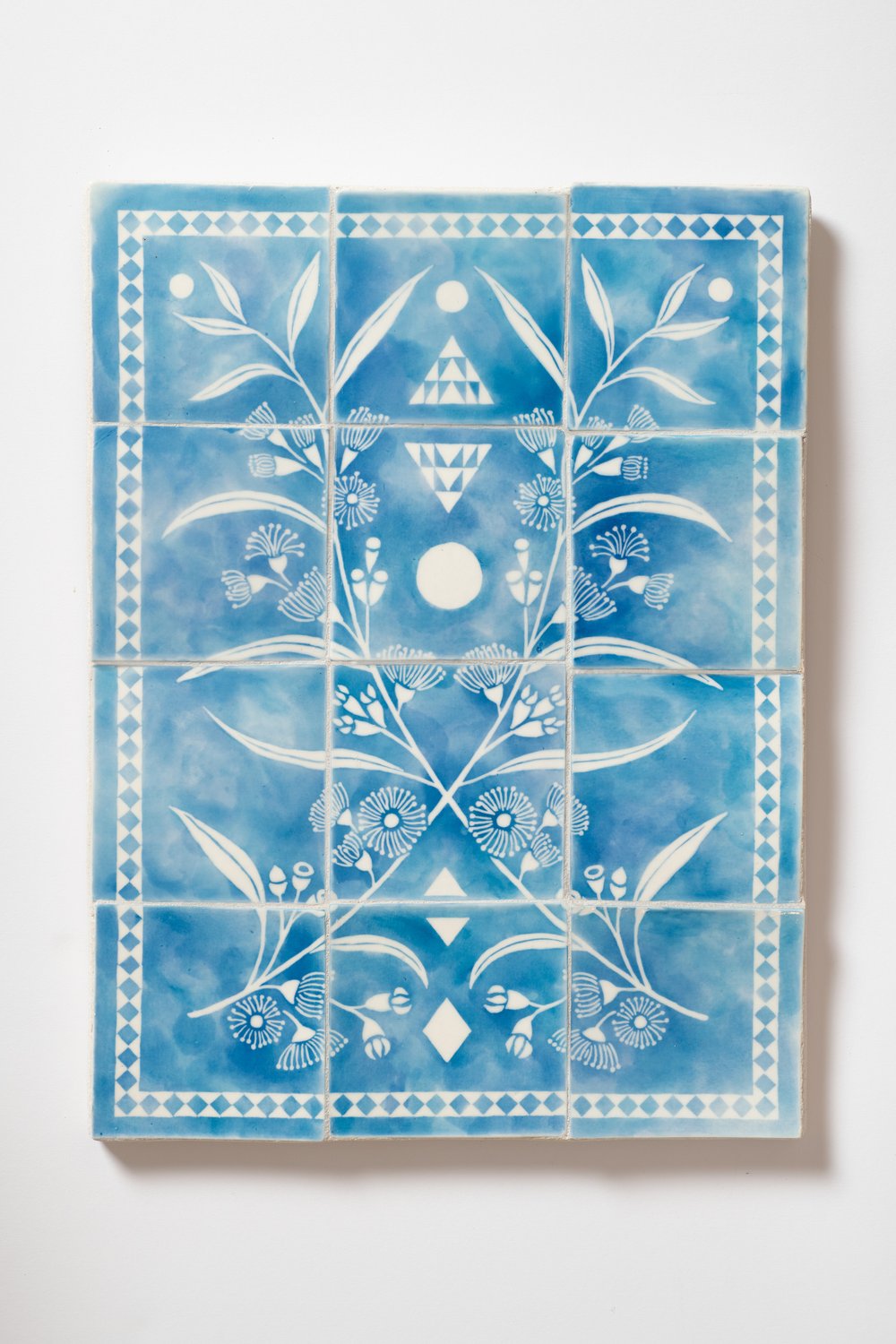The image is a vertically-oriented photograph with an off-white to light beige gradient background, slightly darker at the bottom and fading upwards. In the center, there is a rectangular arrangement of 12 blue ceramic tiles, aligned in a 3 by 4 grid. The tiles, resembling a dark periwinkle blue, are slightly unevenly aligned, giving the impression of a puzzle or mosaic pieced together. Each tile features intricate white designs, including circles, diamonds, floral patterns, stems, and leaves. Surrounding the tiles is a white border decorated with blue diamond shapes, adding a decorative frame to the composition. The overall color palette is a gradient blend of blues and whites, with no text present in the image.